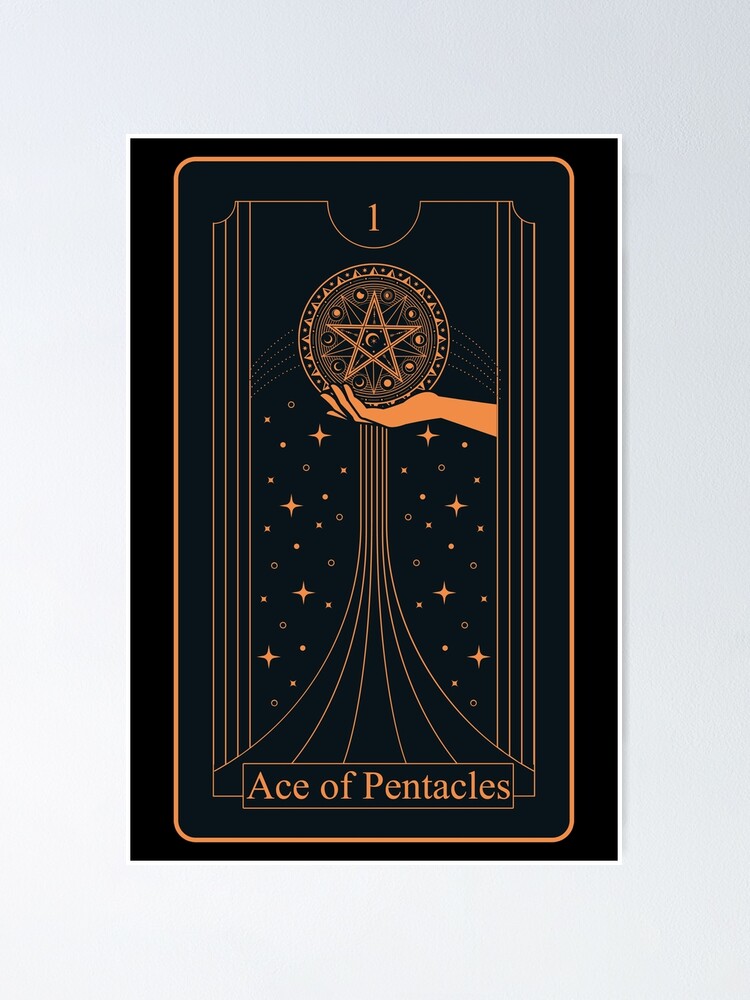The image depicts a tarot card titled "Ace of Pentacles." The card features a predominantly light blue background with a gold border that frames the central illustration. In the center, a hand reaches down from a cloud near the top of the card, holding a single gold pentacle adorned with various star motifs. Above the pentacle, the number "1" is clearly visible. Below the hand, a field with five green hills and a winding path stretches upward towards the hand. The bottom of the card includes text that reads "Ace of Pentacles" in gold. Surrounding the central image, there are small peach and orange stars, adding an additional decorative element. The entire design is reminiscent of a card used in fortune telling or divination practices.